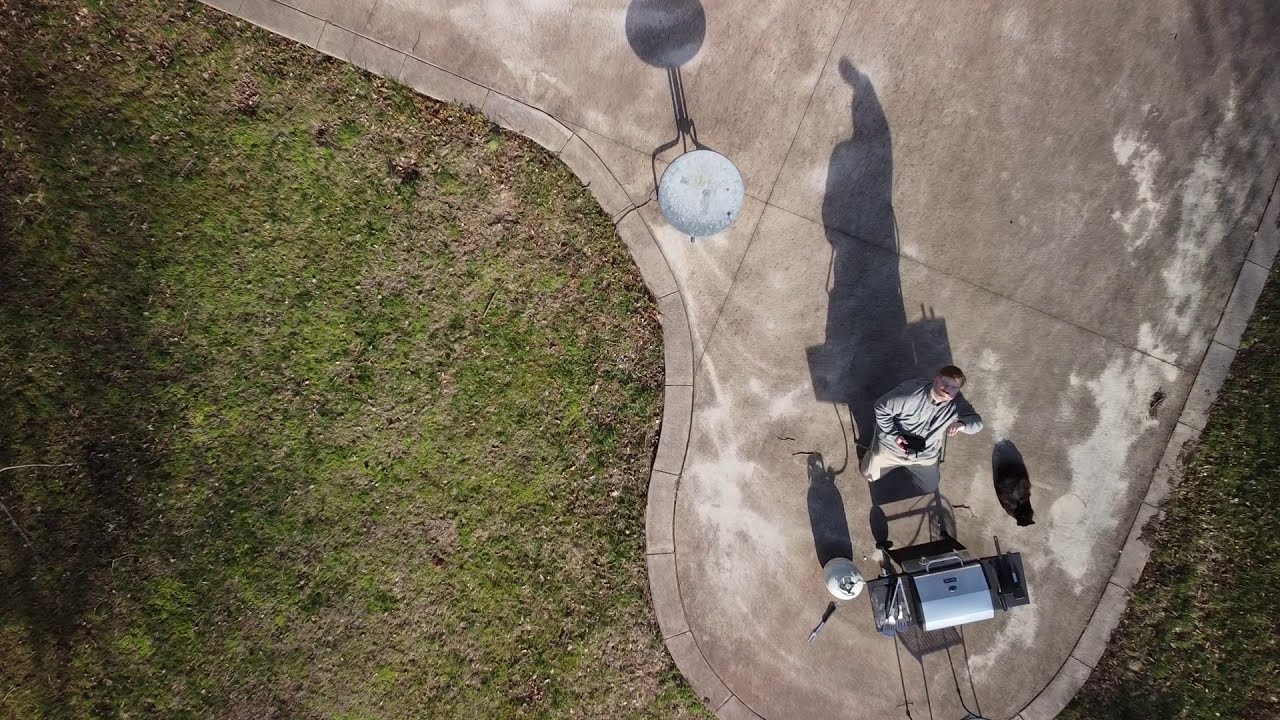This is an aerial daytime photograph capturing a man standing on a concrete patio, likely taken with a drone that he is operating. The man, with short reddish hair, is wearing a gray shirt or sweatshirt and light-colored pants, potentially khakis. He has a mustache and may be wearing glasses. He holds a black device, presumably the drone's remote control, in front of him, casting a shadow on his face. Nearby on the patio is a silver-topped grill, which might be either gas or charcoal, and a small round table behind him. At his feet, a black cat lies on the ground. The patio, which forms an arch-shaped apron, is bordered by grass and scattered leaves, contributing a green and brown hue to the scene. The concrete appears wet, suggesting recent rain. Shadows of the man, the grill, and possibly other objects are visible on the patio surface.